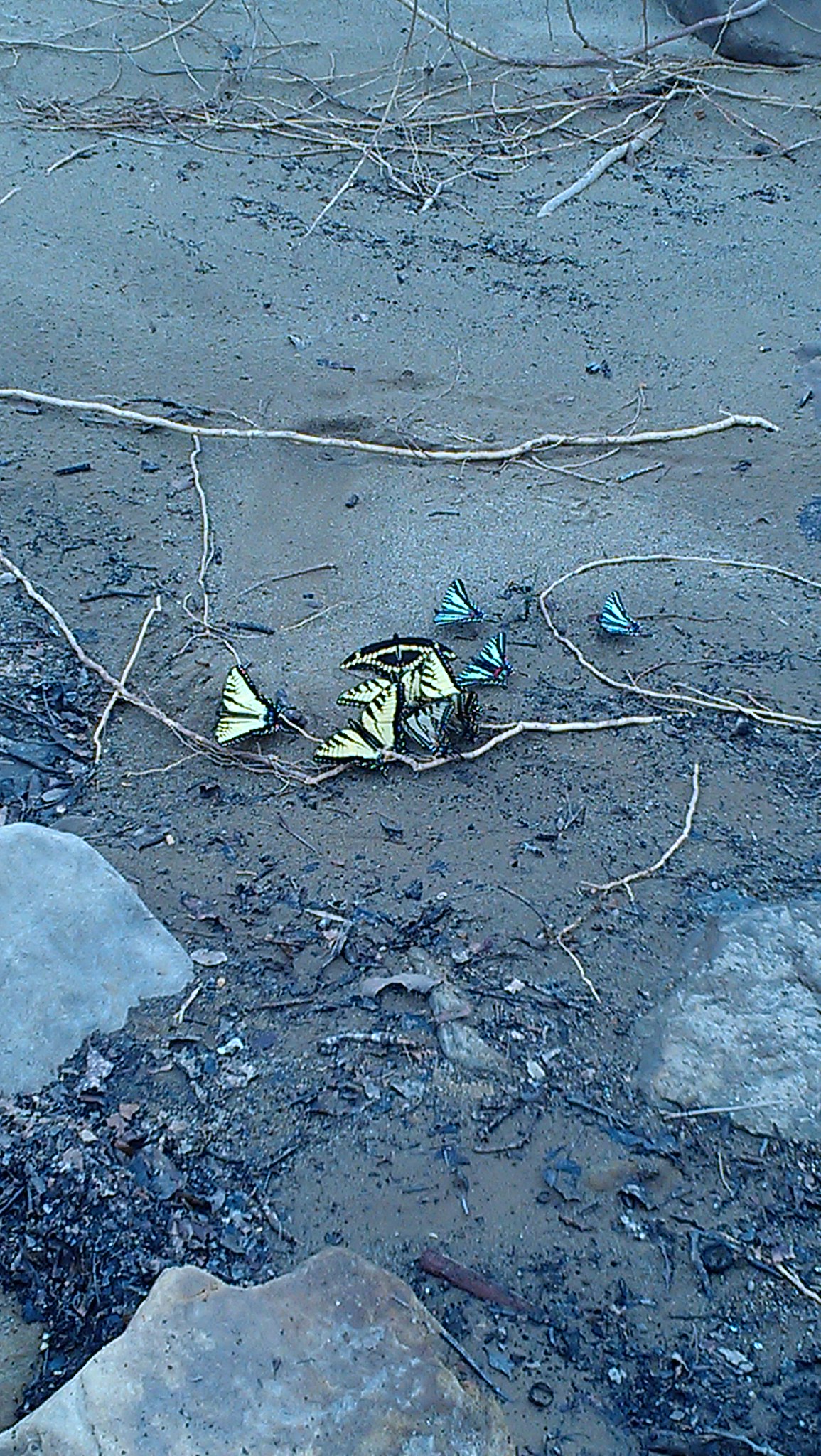This color photograph, taken outdoors, captures a patch of muddy, rocky ground following a recent rainstorm, evidenced by the scattered rock litter and broken branches. The foreground features three large stones with a light blue shimmer, adding a bluish cast to the photo, which contrasts with the naturalistic colors. The central focus of the image is a dried, dead branch embedded in the soil, adorned with about eight small butterflies. These butterflies, predominantly yellow and black with a few smaller white and black ones, appear to be drinking water from the mud, their proboscises extended into the soil. Some butterflies also perch on the branch, creating a scene that initially suggests blossoms due to their vibrant wing patterns. Surrounding the main branch, additional twigs and branches further illustrate the aftermath of the storm. This photograph intricately showcases the resilience of nature amid debris, emphasizing the butterflies' delicate beauty against the rugged, storm-affected landscape.